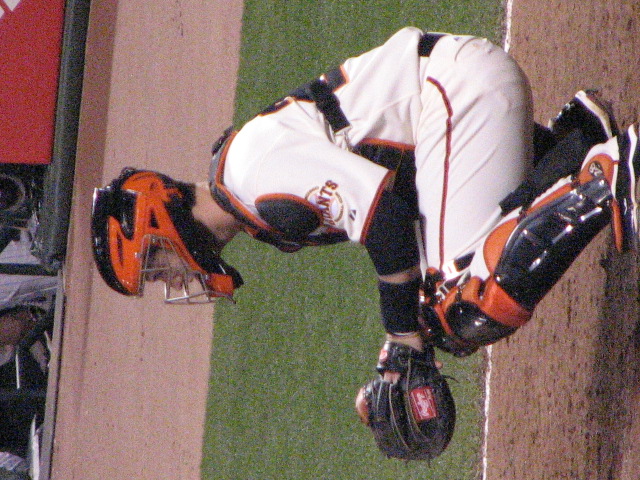The image captures a detailed side profile of baseball catcher Buster Posey in his familiar squatting position, ready to catch the ball. Posey, in his recognizable San Francisco Giants uniform, sports the team's colors: a white uniform with black and orange protective gear, including shin guards bearing the number 28. His distinct black glove is visible on his left hand. The helmet, colored orange and black, is another identifier. The sleeve of his uniform partially displays the word "Giants." Behind Posey, the background reveals the ball field featuring patches of dirt and green grass, with a batting cage and other players distantly visible. The overall scene suggests an authentic in-game moment, likely in an outdoor stadium.